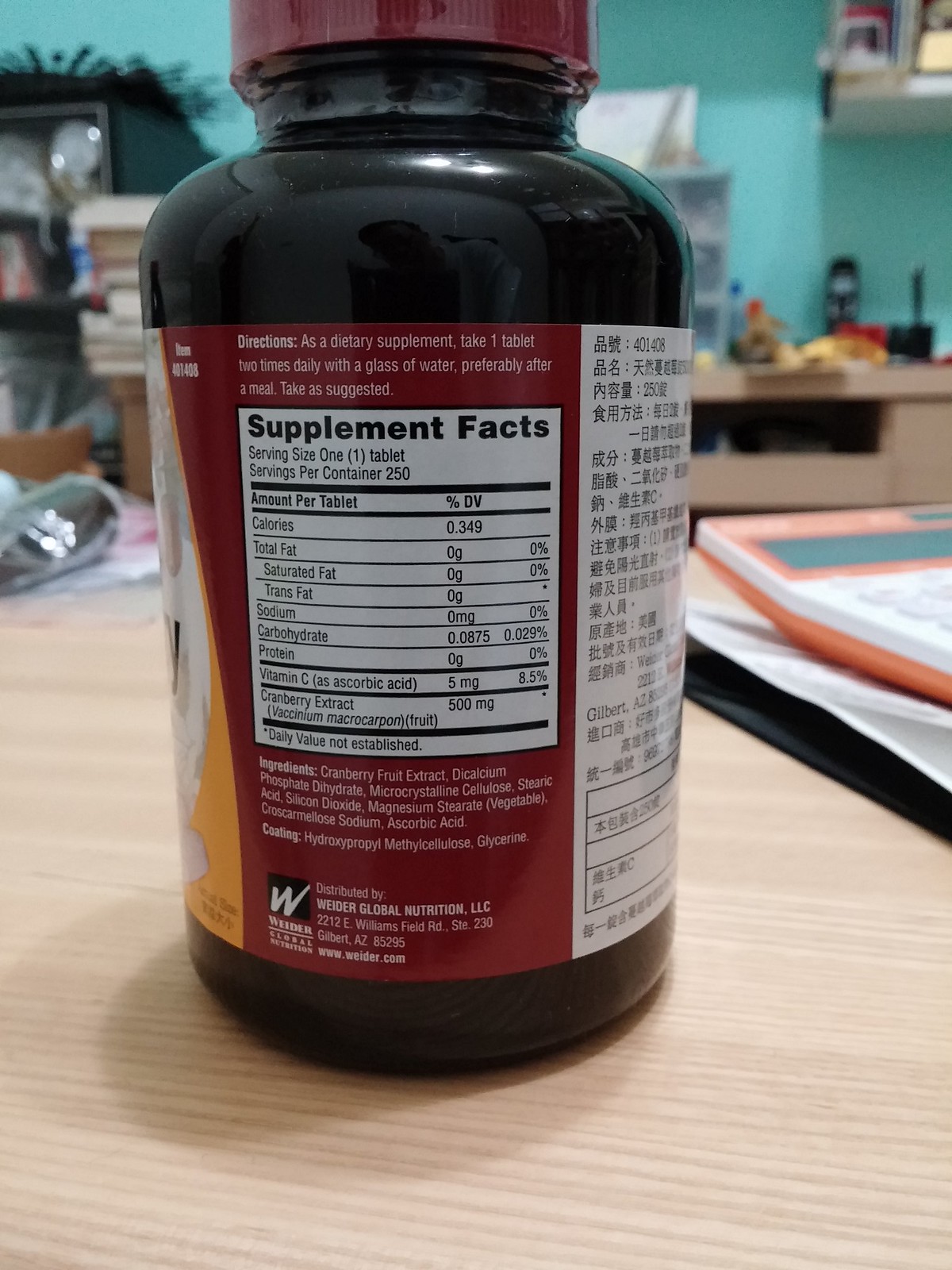In the foreground of the image, there is a bottle of dietary supplement prominently displayed. The label facing forward provides detailed nutritional information. This particular supplement is cranberry extract, containing 500 milligrams of the extract per tablet, also providing the Latin name, Vaccinium macrocarpon. 

The nutritional details are meticulously listed: each tablet has 0.349 calories, zero grams of total fat, saturated fat, and trans fat, zero milligrams of sodium, 0.0875 grams of carbohydrates (0.029% of the daily value), zero grams of protein, and five milligrams of vitamin C. The ingredient list includes cranberry fruit extract, dicalcium phosphate dihydrate, microcrystalline cellulose, stearic acids, silicon dioxide, vegetable-sourced magnesium stearate, a form of sodium, and ascorbic acid. The tablet's coating is made from hydroxypropyl methylcellulose and glycerin. The supplement is manufactured by Whiter Global Nutrition LLC, based in Gilbert, Arizona.

In the background, the setting appears to be an office with a pale bluish-green wall. A phone and a shelf with assorted items are visible along with an orange and white calculator to the right of the bottle, adding context to the scene. The mixed languages on the bottle include English and possibly Japanese, Korean, or Chinese script, enhancing the global appeal and utility of the product.